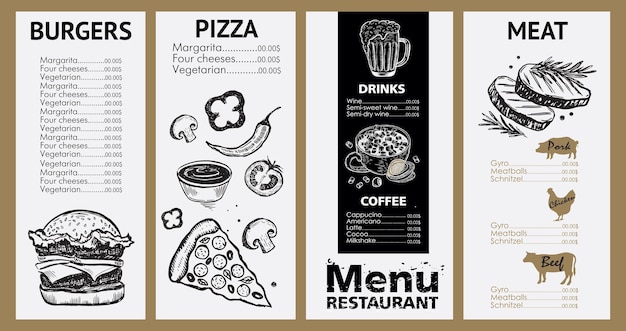The image depicts a placeholder restaurant menu template, divided into four vertical sections on a tan background with a brown border. Each section features black and white illustrations and placeholder text.

1. **Burgers**:
   - This section has the header "Burgers" at the top. Under it, listed repeatedly, are the burger types: "Margherita," "Four Cheeses," and "Vegetarian." Each is shown multiple times. At the bottom, there is a graphite drawing of a cheeseburger with a seeded bun, lettuce, and cheese.
   
2. **Pizza**:
   - The "Pizza" section also lists "Margherita," "Four Cheeses," and "Vegetarian." Beneath the text, there are black and white drawings of pizza toppings, including a mushroom, a tomato slice, a hot pepper, a ring of green pepper, a tub of sauce, and a slice of pizza.

3. **Drinks**:
   - This section starts with "Drinks" and lists the items: "Wine," "Semi-sweet Wine," "Semi-dry Wine." Below these, it lists coffee variants: "Coffee," "Cappuccino," "Americano," "Latte," "Cocoa," and "Milkshake." There are pen and ink drawings of a beer pitcher and a coffee cup. Additionally, this panel includes the words "Menu" and "Restaurant."

4. **Meat**:
   - The final section titled "Meat" lists different types of meat dishes: "Pork," "Gyro," "Meatballs," "Schnitzel"; the same pattern repeats for "Chicken" and "Beef." Each type is paired with a silhouette of the respective animal: a pig for pork, a chicken for chicken, and a cow for beef. There are also drawings of steaks with sprigs of rosemary.

Overall, the menu features placeholder names and zero-dollar prices, indicating it is a template yet to be customized.